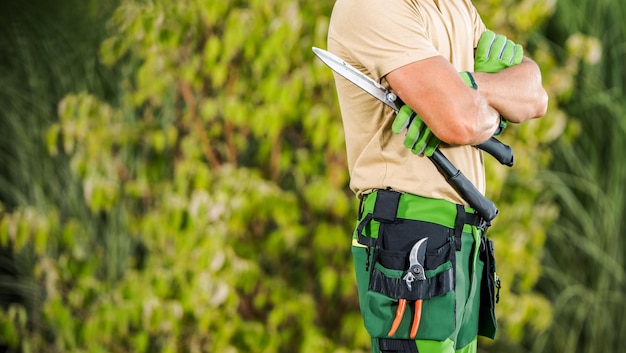In this detailed landscape-oriented color photograph, a male individual is the central subject, depicted from the top of his shoulders to just below his hips. He stands upright, facing right, with his arms crossed over his chest, illustrating a confident and relaxed posture. He is dressed in gardening attire, featuring a light tan short-sleeved shirt and green pants. His bright green latex gloves draw attention, complementing his outdoor work theme.

Under his right arm at the elbow, he holds a large pair of gardening shears with long, black handles forming a V shape and pointed silver blades, evidencing his readiness for gardening tasks. A green tool belt or waistband accessorizes his outfit, contributing to an organized appearance. Attached to the belt, near his right hip, is a smaller pair of pruning shears with distinctive orange handles and a silver arced blade.

The background consists of lush greenery, including plants, trees, and bushes, providing a natural and serene ambiance. The foliage is slightly blurred, enhancing the focus on the subject while indicating a daytime outdoor setting through the brightness of the scene. This photograph embodies a realistic and representational look, capturing the essence of a gardener amidst his natural environment.